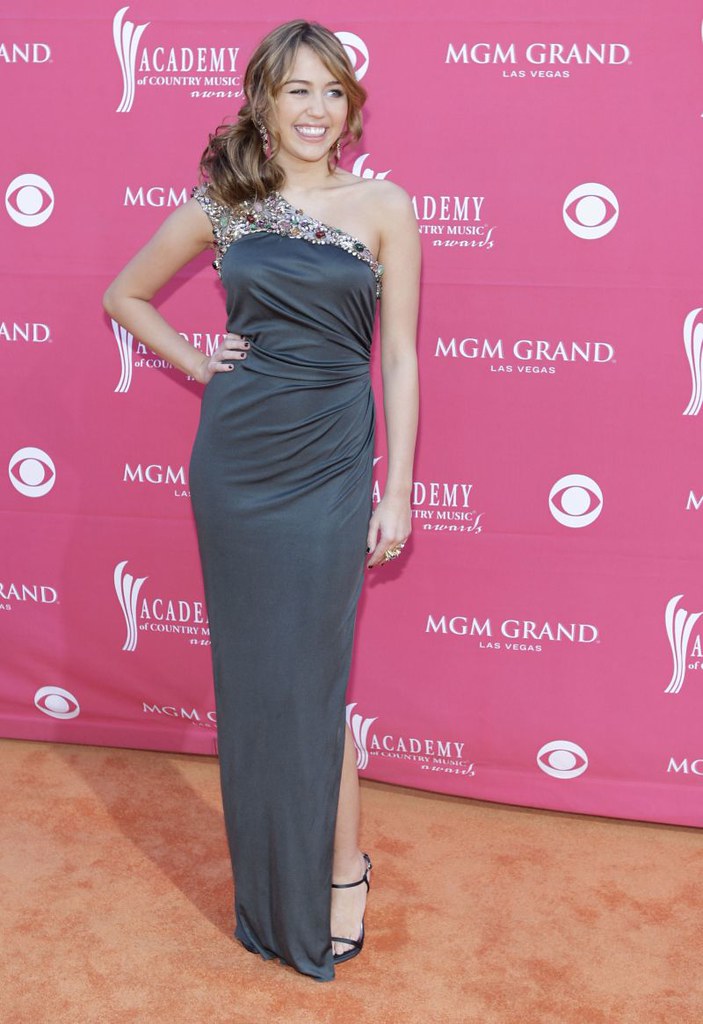In this Getty image captured approximately a decade ago, Miley Cyrus is at an event, likely the Academy of Country Music Awards, taking place at the MGM Grand in Las Vegas. She is elegantly posed on a pinkish-beige carpet against a pink backdrop adorned with white logos for MGM Grand Las Vegas and the Academy of Country Music. Miley is dressed in a striking gray one-strap gown embellished with encrusted jewels on the left side of the strap. Her hair is styled in a side ponytail and she sports a radiant smile at the camera. Additional details include her painted nails, rings, and heeled shoes. The image captures her standing outside in the center, exuding confidence and glamour amidst the event's sponsors.